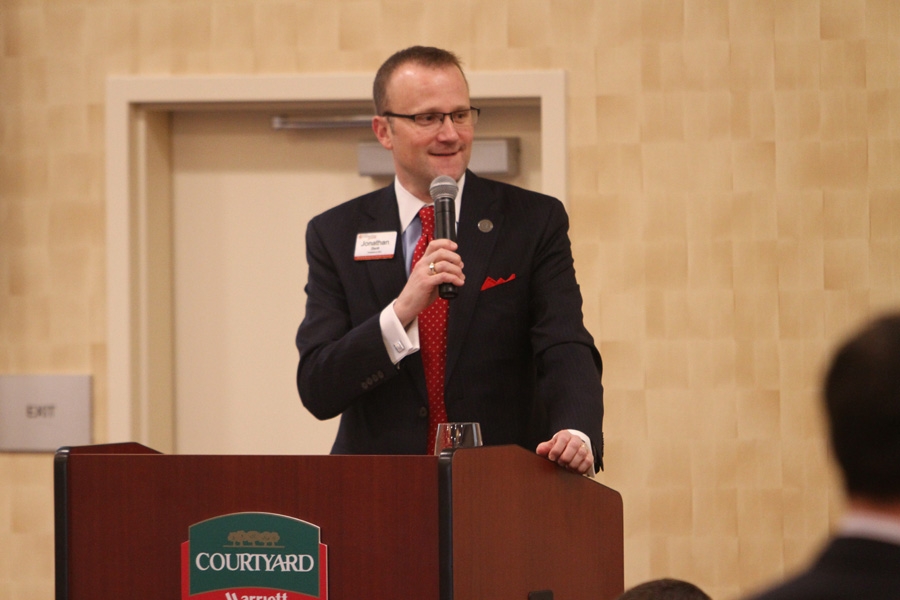In the photo, a man in his mid-30s with glasses and receding short hair is captured mid-speech behind a large, brown wooden podium. He is holding a microphone close to his mouth, looking to his left with one hand resting on the podium. Dressed in a formal black suit, he also sports a red tie with white polka dots, a white-collared shirt, and a red handkerchief peeking from his pocket. A white name tag is visible on his jacket. In front of him, a clear glass with a drink sits on the podium.

The podium bears the word "Courtyard" in white letters with green borders, above a red section featuring the word "Marriott" and an illustration of green trees. The background consists of a beige checker-patterned wall with a closed door visible behind him. The setting appears to be a large room, perhaps a conference hall, evidenced by the blurred head of a person in the foreground, indicating he is speaking to a large audience.